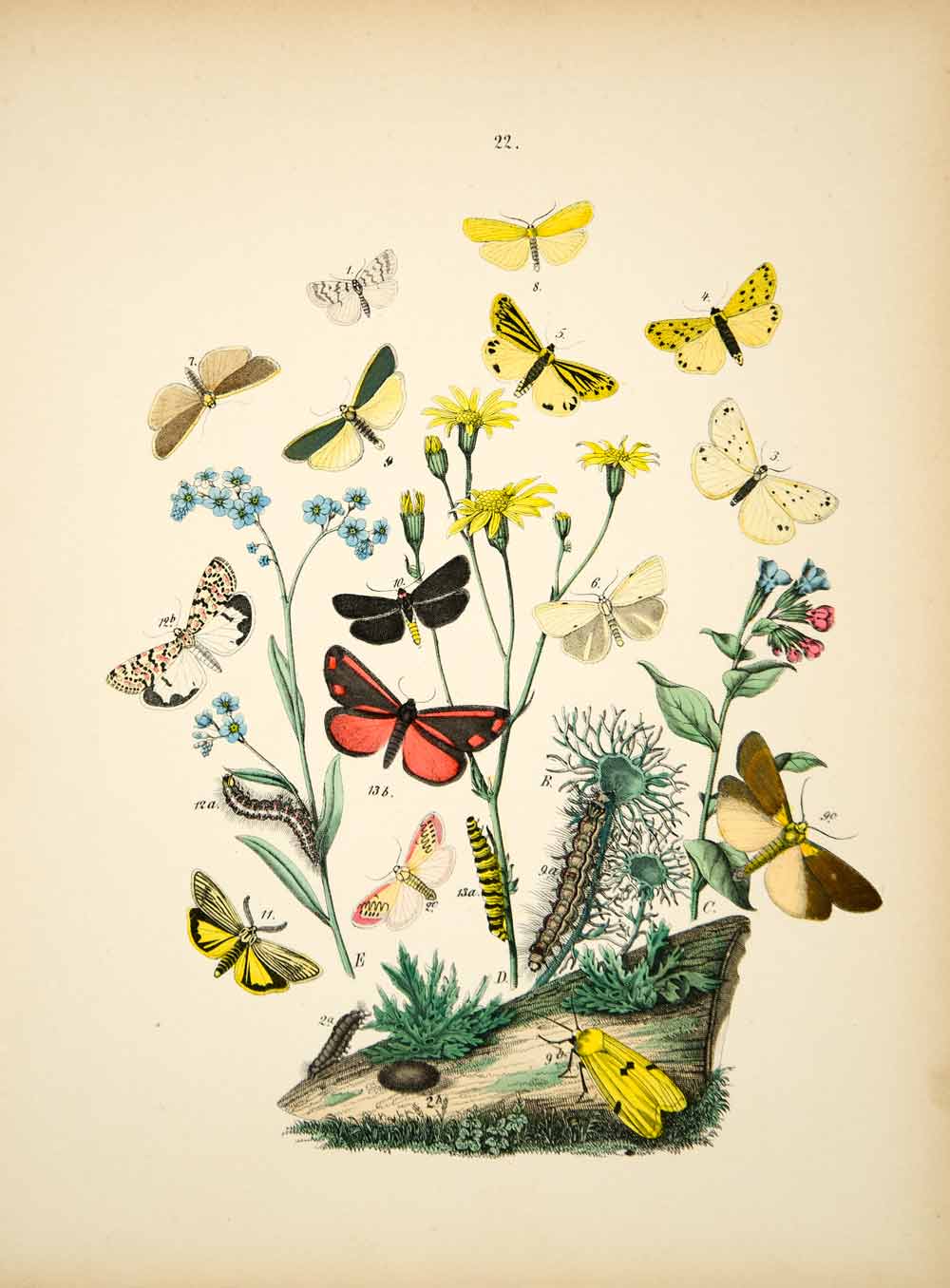This detailed drawing, set against a cream-colored background tinged with pink, showcases a diverse range of butterflies and insects in various life stages, likely from an old botanical and butterfly collection book. The butterflies, numbering from 1 to 22, are illustrated in soft pastel shades, predominantly smooth yellows and greens. Each butterfly is uniquely colored and patterned, with some displaying yellow hues while others boast red, black, or spotted designs.

Amidst these butterflies are several plant stalks supporting different insects. One stalk features a white and black caterpillar, another is adorned with red and blue flowers, and yet another has a brown caterpillar possibly in flight. At the bottom of the image, a piece of driftwood or regular wood holds a yellow butterfly with its wings closed.

The overall scene is teeming with life, featuring not just butterflies but also ladybugs, and various caterpillars, all meticulously numbered and classified, suggesting a scientific or educational purpose. The illustration is vibrant yet subdued, avoiding any bright colors, and evokes a sense of careful observation typical of historical naturalist documentation.